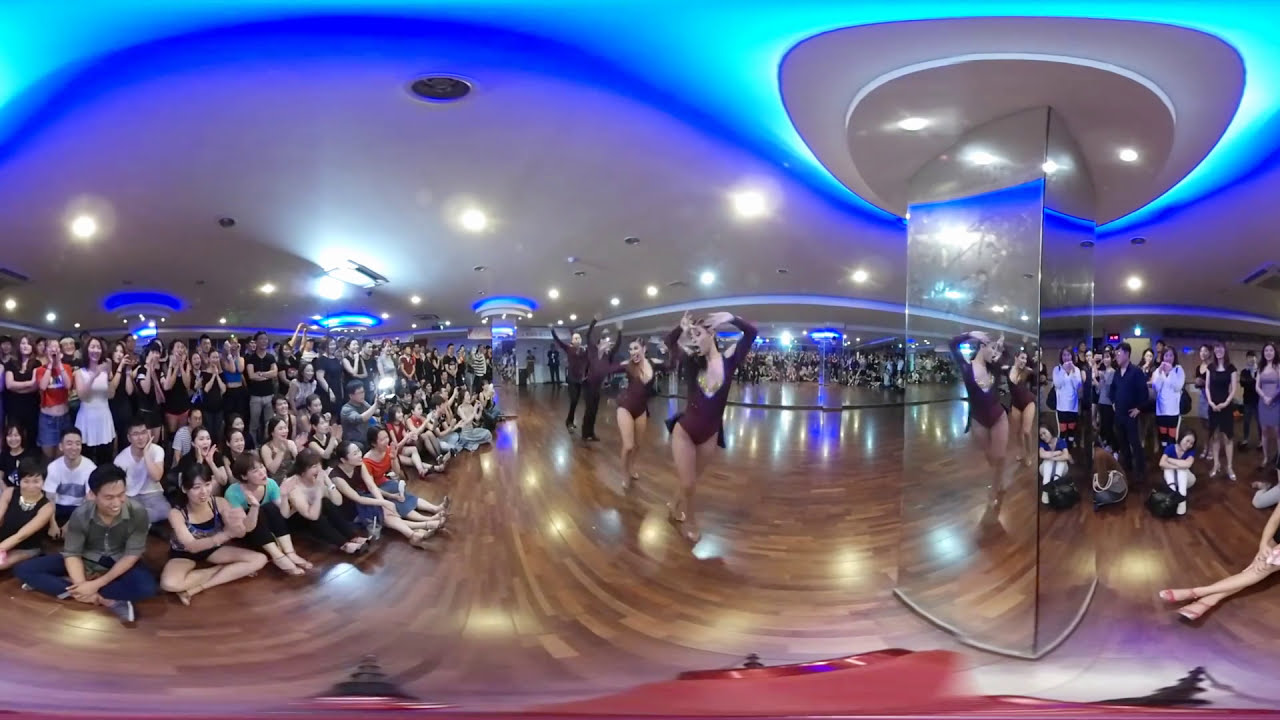This panoramic image captures a lively scene inside a large dance studio with glossy, multi-colored brown hardwood floors and an array of mirrors. The central focus is on four dancers performing elaborate ballet or salsa movements. Two men, dressed in maroon shirts and black pants, are poised behind two women clad in matching long-sleeve maroon leotards. They are surrounded by a crowd of onlookers: the front rows are seated cross-legged, taking photos, while those behind stand attentively. A reflective, multi-sided mirror column stands on the right, with a ceiling above adorned with curved patterns of dark and light blue accent lights along with multiple small circular white fixtures. The composition appears slightly distorted due to the panoramic photograph effect, bending people and objects into a dynamic, almost surreal scene.